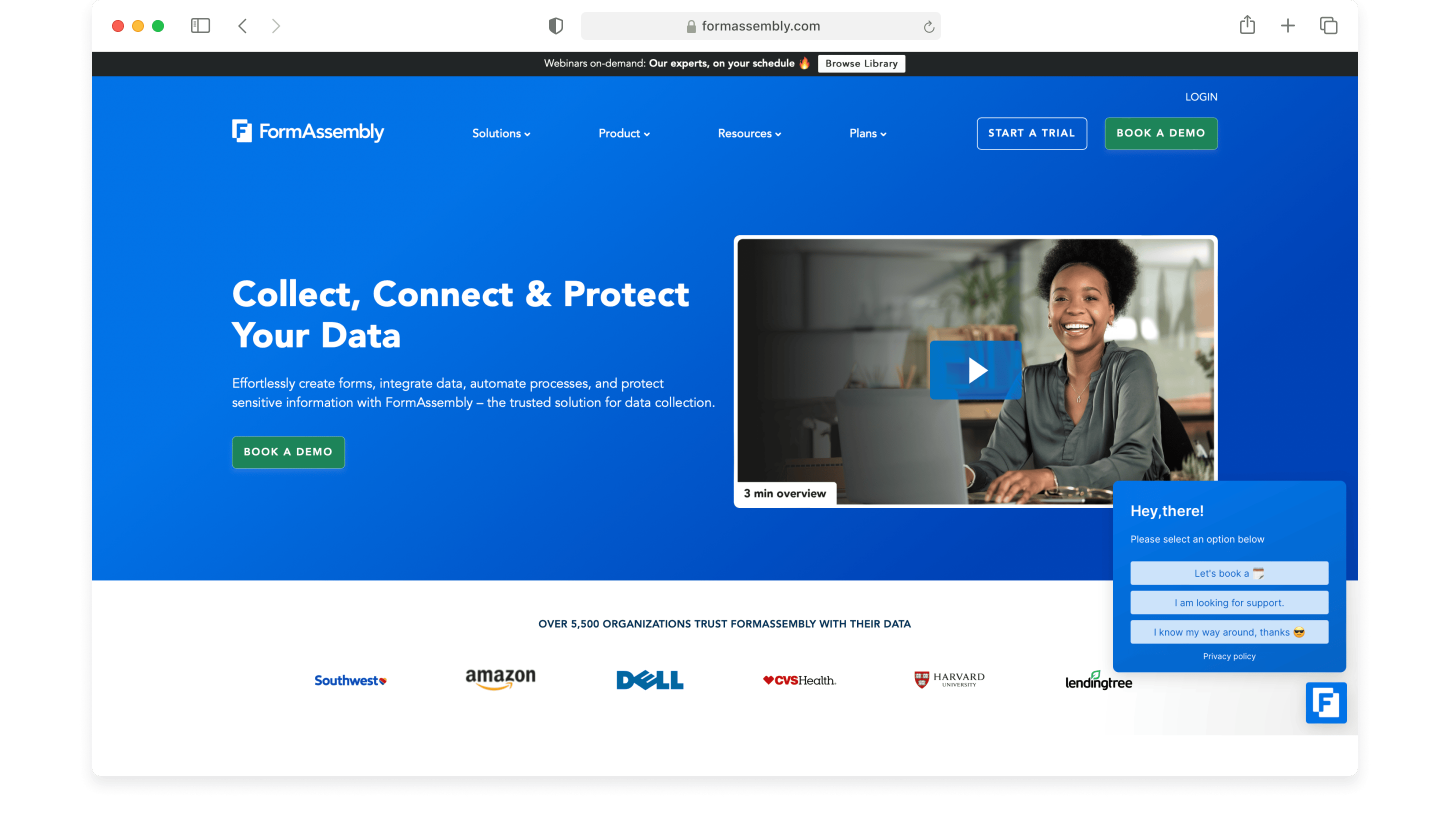This image captures a detailed view of the FormAssembly website. At the top center, the URL is visible, flanked by a set of icons on the left, including red, yellow, and green dots in the top-left corner. On the right, three computer-related icons are present. Beneath this is a black bar, followed by a predominantly blue screen which prominently displays "FormAssembly."

The screen features four categories in white text, a blue button labeled "Start a Trial," and a green rectangular button labeled "Book a Demo" in white text to the right. Above these is an option to log in. Below, on the left, there's a section with the phrases "Collect, connect, and protect your data" in white, accompanied by a smaller, hard-to-read sentence beneath it. There’s also another green "Book a Demo" button.

A square image showcases a tutorial video featuring a play icon in its blue center. The individual in the video, who has darker skin tone, black hair, and is wearing a gray shirt, is smiling while using a computer. This scene is set against a gray background adorned with a few houseplants. 

In the bottom right corner of the image, there’s a chat widget with "Hey there" followed by some small text and three small, unreadable options within a light gray rectangle. Adjacent to this is a blue square bearing a white "F" at the center. At the footer of the image, text reads "Over 5,000 organizations trust us with their data," followed by logos of six well-known brands.